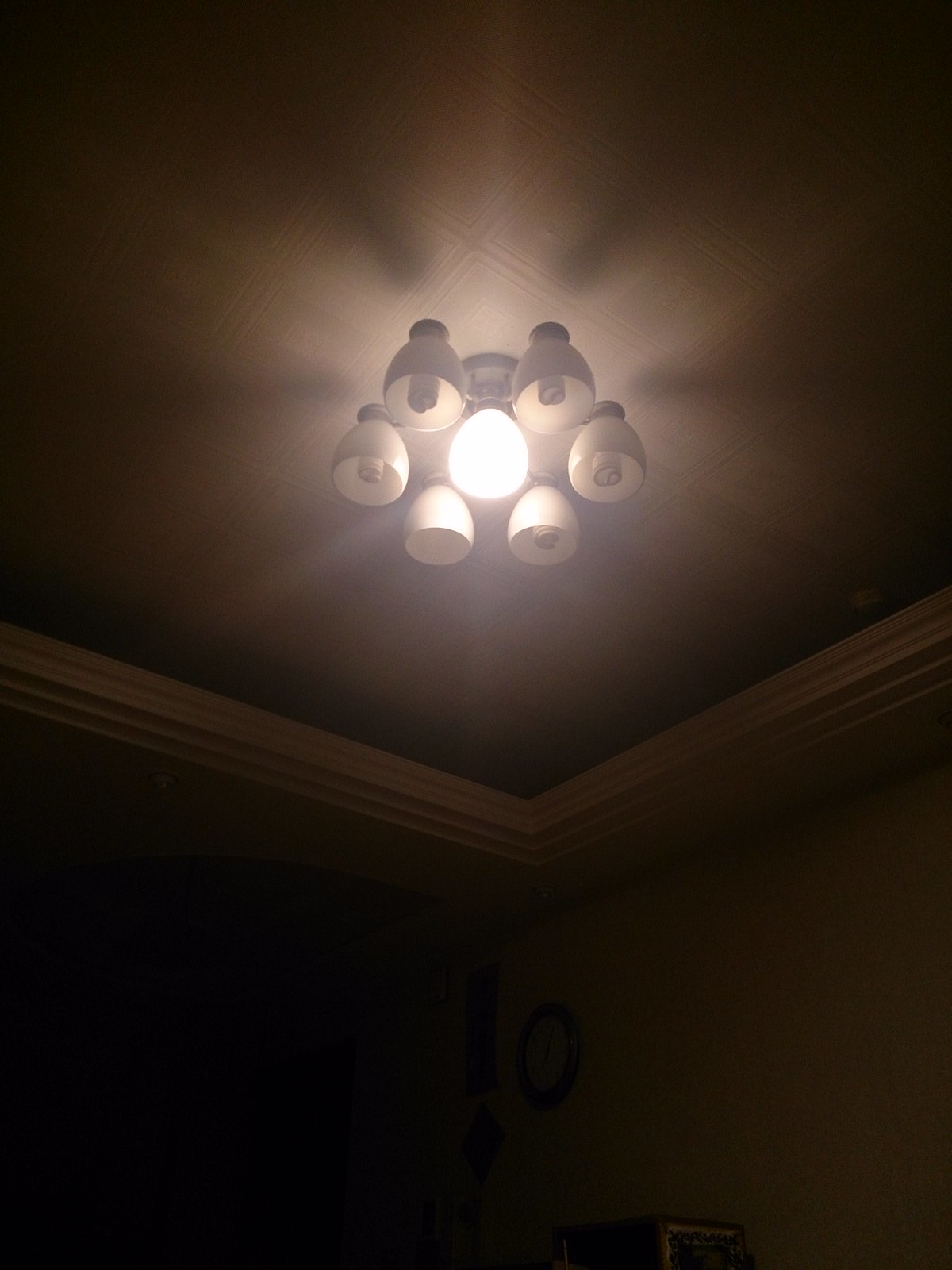The image depicts a dimly lit interior room with two visible walls meeting at a corner. The walls are a mixture of dark colors, with the left wall appearing almost black and the right wall in a tannish brown. Crown molding, light brown in color, accentuates the top of the room where the walls meet the ceiling. 

The ceiling features a pattern of squares reminiscent of an old-fashioned tin ceiling, giving it a textured but not deeply creviced appearance. Dominating the ceiling is an illuminated light fixture with a central globe emitting bright white light, which creates a snowflake-like pattern of rays across the ceiling. Surrounding this central globe are six smaller globes, each containing compact fluorescent light bulbs that are currently turned off.

On the wall, there's a dark circular object, possibly a clock, alongside another indistinct object positioned slightly below it. Despite the central illumination, the room remains quite dark, with the light failing to extend much beyond the upper sections of the walls, leaving the lower part of the room in shadow.